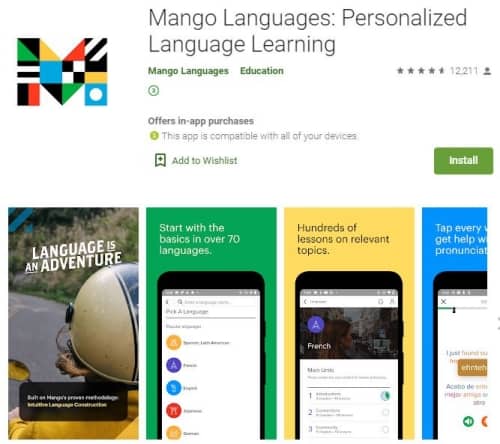The image features a white background with a vibrant, multi-colored "M" at the top, showcasing stripes, squares, and dots in green, blue, black, white, red, and yellow hues. Beneath the "M," the text reads "Mango Languages, personalized language learning." Further down, it lists "Manage Languages, Education," accompanied by a four-and-a-half-star rating. A small circle with an "i" inside indicates additional information, and another small yellow circle signals the availability of in-app purchases. The text mentions that the app is compatible with all your devices. A small square featuring a plus sign reads "Add to Wishlist," followed by a prominent green "Install" button.

Below these elements are four separate boxes with images and text. The first box, featuring an adventurous individual wearing a helmet near a river, is captioned "Language is an adventure." The second, a green box with a phone background, states, "Start with the basics in over 70 languages." The third, a yellow box also with a phone background, proclaims, "Hundreds of lessons on relevant topics." The fourth, a blue box partially cut off, hints at helping with pronunciation skills.